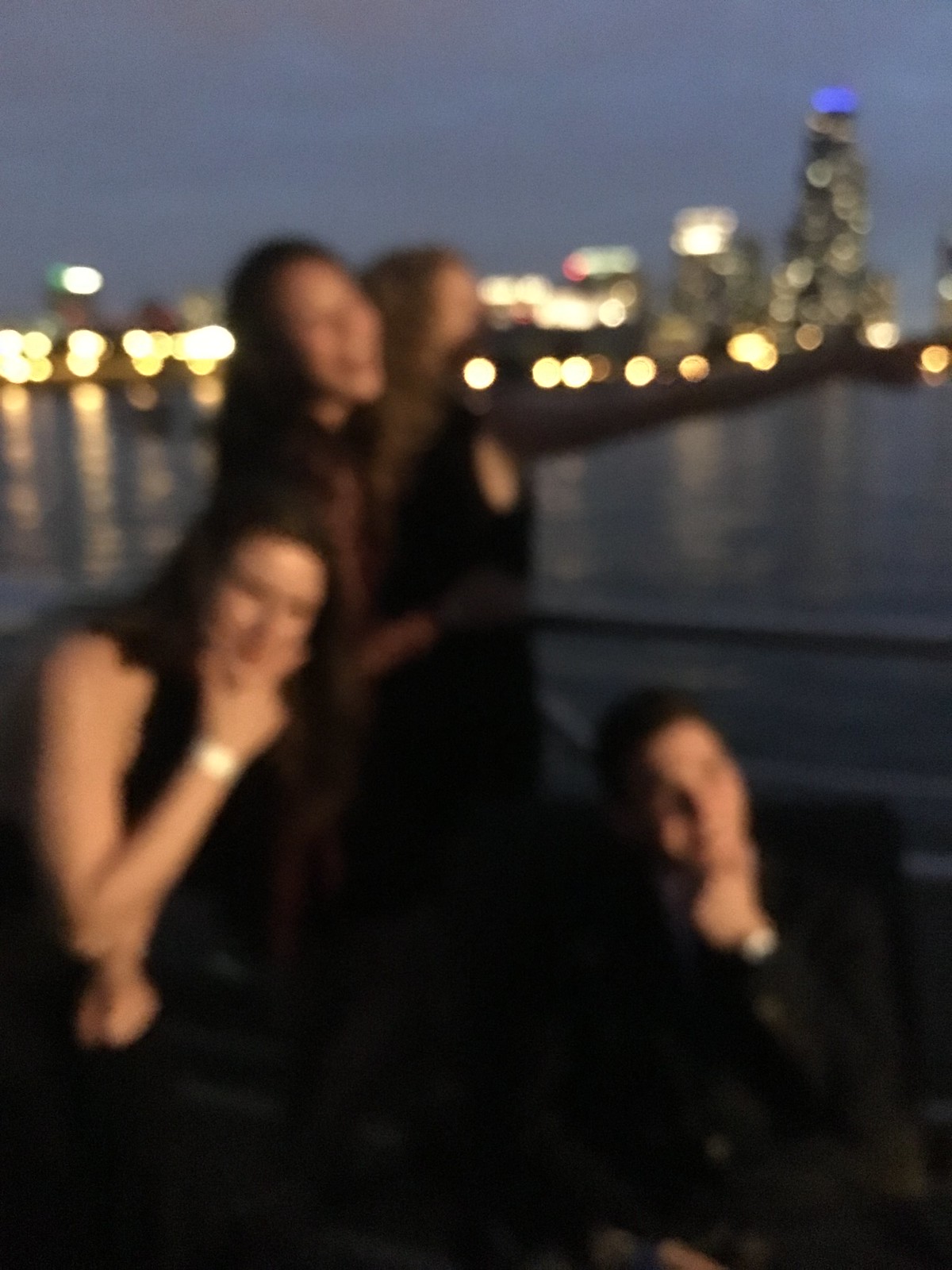In this blurry nighttime photograph, four individuals—two men and two women—are dressed in what appears to be formal attire as they pose outside by a waterfront. The cityscape in the background glows with building lights, including a prominent tall building with blue lights at its peak. The night sky features a murky blue hue, punctuated by the soft glow of yellow orbs from the urban lighting. The image's lack of clarity obscures specific details about the attire, but all four seem to be wearing dark, possibly black, clothing. In the foreground, a man stands on the right and a woman on the left; both are seen holding their hands near their chins, with the woman forming a 'V' shape with her thumb and forefinger. Behind them, two other women with long brown hair stand, completing the group. A railing separates them from the water, adding a sense of depth to this otherwise indistinct, yet atmospherically rich scene.